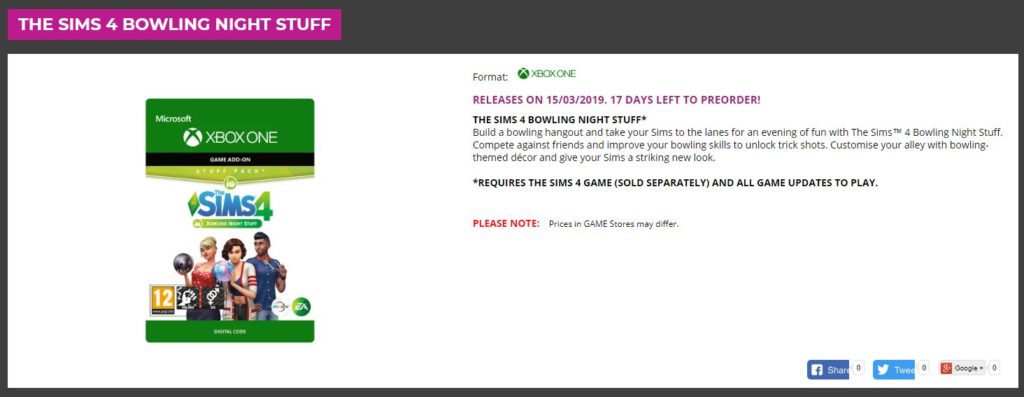The image features a detailed promotional layout for "The Sims 4: Bowling Night Stuff" game add-on for Xbox One. The border of the image is gray, and the top part boasts a vibrant magenta rectangle with the text "The Sims 4: Bowling Night Stuff" in white.

In the main section, the background is predominantly white. Towards the left side, the cover design is presented, which is green. At the top of this cover, "Microsoft" is written in white, followed by "Xbox One" in white text below it. Underneath, there is a black border with the words "Game Add-On" in white. The title "The Sims" is displayed in blue, with the number "4" in green beside it. The cover also prominently features three animated characters, two of whom are holding bowling balls, signifying the bowling theme of the add-on.

On the right side of the image, various important details are listed: 
- The text "Xbox One" in green stands out against a black background.
- In magenta, it states "Releases on 15/03/2019, 7 days left to pre-order."
- In bold black text, the main title "The Sims 4: Bowling Night Stuff" is reiterated along with accolades.

A descriptive paragraph in black reads: 
"Build a bowling hangout and take your Sims to the lanes for an evening of fun with The Sims 4: Bowling Night Stuff. Compete against friends and improve your bowling skills to unlock trick shots. Customize your alley with bowling-themed decor and give your Sims a striking new look." 

Important notes follow in bold black text: 
"Requires The Sims 4 game (sold separately) and all game updates to play" (in all caps). 

Below this, in bold red text:
"PLEASE NOTE" (in all caps).

Finally, in standard black text:
"Prices in-game stores may differ."